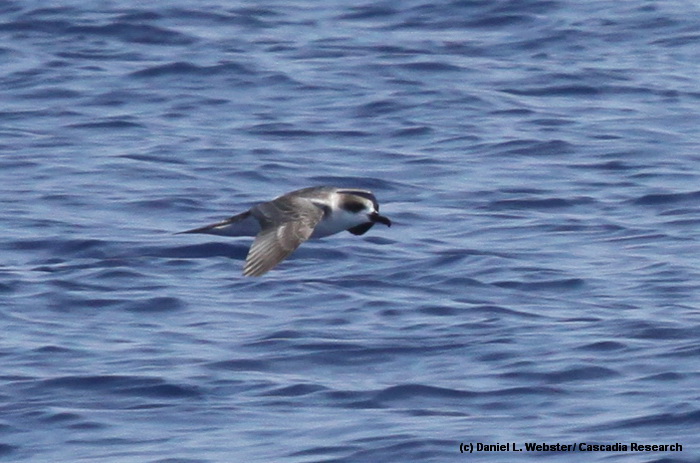A stunning photograph captures a graceful gull in mid-flight over a slightly choppy expanse of blue water. The bird's predominantly gray plumage contrasts beautifully with its pristine white underbelly, while dark gray or black markings highlight its eyes, and a sleek black beak adds a touch of elegance. The subtle movement in the water below complements the dynamic pose of the bird, creating a sense of motion and freedom. A black printed watermark in the bottom right corner credits the photographer, Daniel L. Webster, with the inscription "Cascadia Research."